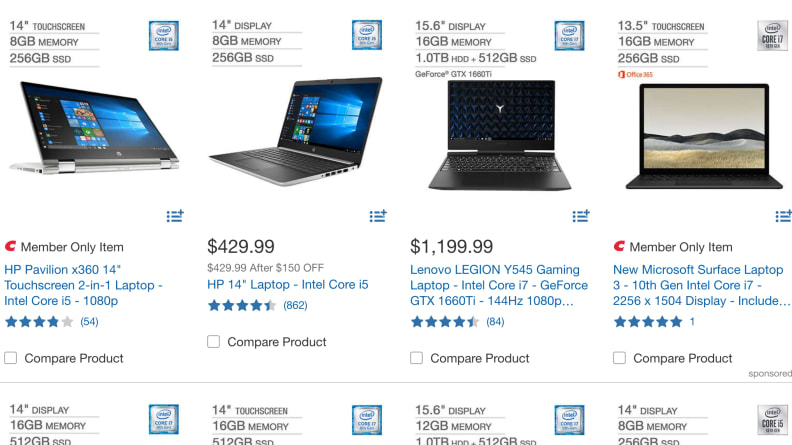The image depicts a section of an e-commerce website displaying a selection of laptops available for purchase. The layout features four columns and two rows, although the bottom row is partially truncated, showing only the top portion of the items.

Starting from the left in the top row:

1. The first laptop is the **HP Pavilion X360 14-inch 2-in-1 Laptop** with a versatile screen that can rotate 360 degrees to lie flat against the back of the keyboard. It boasts a 14-inch touch screen, 8GB of memory, and a 256GB SSD. It is an exclusive "Members Only" item, highlighted by a red 'C', and powered by an Intel Core i5-1080p processor.

2. Below this, you find a basic yet efficient **HP 14-inch Laptop** featuring a 14-inch display, 8GB of memory, and a 256GB SSD, priced at $429.99. It is equipped with an Intel Core i5 processor.

3. Moving to the right, the next prominent item is the **Lenovo Legion Y545 Gaming Laptop**, which offers a 15.6-inch display, 16GB of memory, a substantial 1TB HHD along with a 512GB SSD. It is powered by an Intel Core i7 processor and includes a GeForce GTX 1660 Ti graphics card. This gaming laptop boasts a refresh rate of 144Hz and a resolution of 1080p, priced at $1199.99.

4. To the far right, there's the **Microsoft Surface Laptop 3**, with a 13.5-inch touch screen, 16GB of memory, and a 256GB SSD. This model includes Office 365 and is another exclusive "Members Only" item, marked by a red 'C'. It operates on a 10th generation Intel Core i7 processor and displays at a resolution of 2256 x 1504.

The bottom row highlights the top of other laptop selections, hinting at additional options available that are not fully visible in this truncated view.